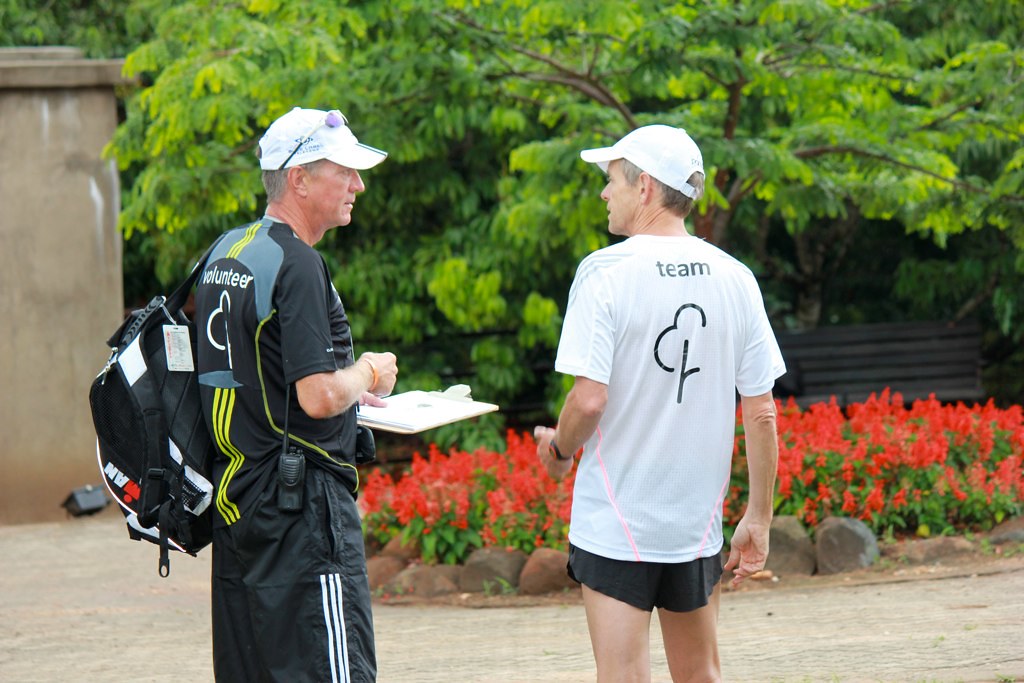In this outdoor daytime photograph, two older Caucasian men stand on a light tan stone walkway, turned slightly inwards towards each other as they converse. The man on the left wears a white ball cap with sunglasses resting atop it, revealing his gray hair. His black short-sleeve t-shirt reads "VOLUNTEER" in white print across the shoulders, complementing his black Adidas sweatpants with white stripes. He carries a black and white backpack over his left shoulder and holds a clipboard in his bent left arm. A walkie-talkie is visible on his right hip. The man to his right also wears a white ball cap and has graying, dark brown hair. He dons a white t-shirt with "TEAM" printed in black on the back and a simplified tree logo below. His black running shorts complete his attire. His left arm is bent, gesturing as he speaks. Between them and the camera, a bed of red fire plants surrounded by brown boulders adds a splash of color. To the left, a stone pillar stands near a wall, while to the right, a large tree shades a black bench. The scene is set in a public garden, with trees visible in the distance, suggesting a peaceful, communal setting in the middle of the day.